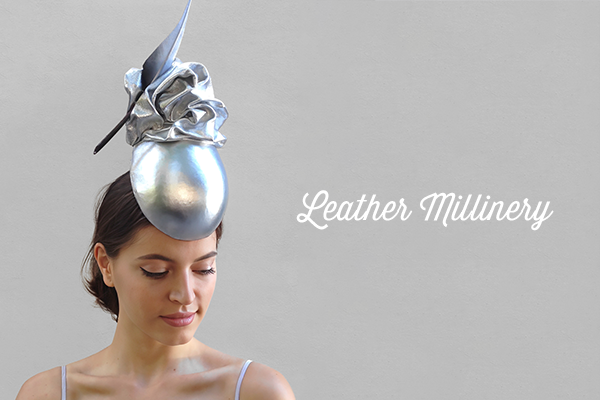In this professionally taken, full-color marketing photograph, a Caucasian woman in her mid-30s is prominently featured against a solid medium gray background. Positioned on the left side of the square image, her shoulders and blue spaghetti straps are visible, suggesting she is dressed in a minimalistic outfit. The woman has short, collar-length dark hair, dark eyebrows, and black eyelashes. Her head is slightly tilted down, with her eyes closed or looking downward, and she wears a light reddish-pink lipstick. Atop her head sits a unique, stylized silver hat. The hat has a prominent silver dome that covers part of her forehead and features a squished silver, leather-like flower with a feather-like object stemming from its left side. The hat is also reflective, capturing light in an eye-catching manner. To the right of the woman, in white cursive text, are the words "Leather Millinery," indicating both the nature of the product and its craftsmanship.